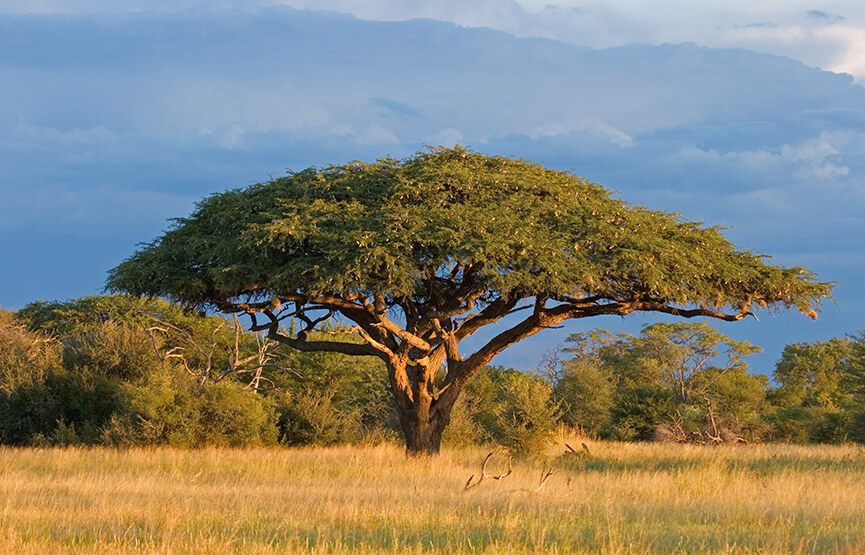This image captures a vast, arid prairie reminiscent of an African savannah. Dominating the scene is a large, umbrella-shaped tree with a thick trunk and a lush, green canopy isolated at the top, devoid of foliage on its lower branches. The landscape is bathed in hues of golden yellow and rich green, indicating a dry yet somehow verdant environment. The foreground features dry, yellowish-green grass interspersed with scattered logs and limbs. Behind the main tree, a line of shrubs and smaller trees stretches across the expanse of the photograph, continuing the sense of openness. The sky above is a mix of deep blue and patches of white clouds, adding depth and a touch of drama to the otherwise serene and expansive setting. The landscape orientation of the photograph encompasses the sprawling nature of the prairie with its wide-open spaces and the central, majestic tree, evoking a scene straight out of a wildlife documentary.